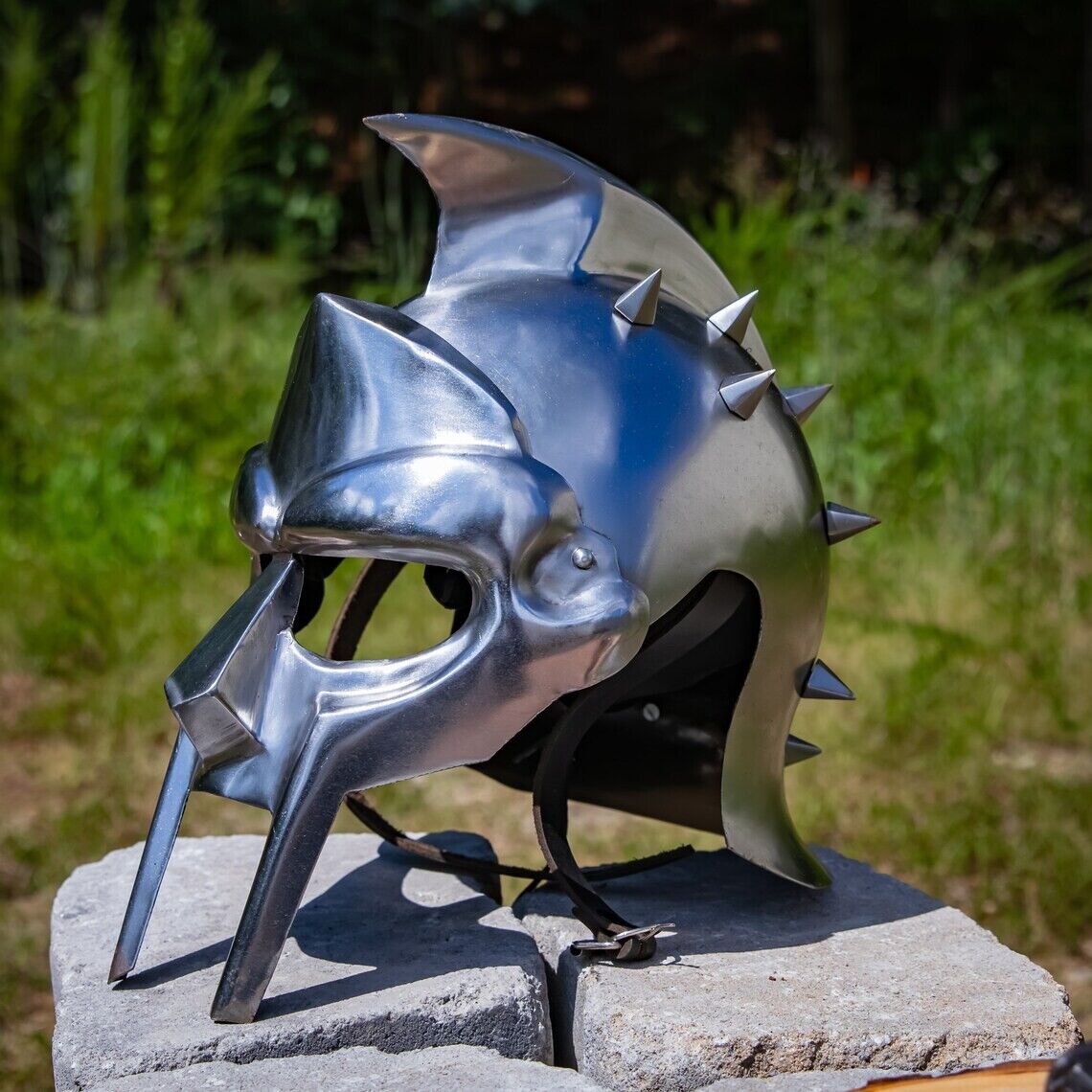The photograph depicts a striking and elaborate silver helmet resting on two gray cinder blocks. The helmet gleams with a slight blue sheen, suggesting a polished metal surface. Designed with clear influences from Roman gladiatorial and Viking styles, the helmet features a prominent crest resembling a mohawk on top, flanked by sharp, pyramidal spikes.

The face mask of the helmet bears a distinct resemblance to a Roman soldier's mask, incorporating angular elements. The eye openings are stark and functional, and a protruding angular nose piece accentuates its fierce demeanor. Extending downward from the face mask are two metal prongs or bars, reminiscent of tusks or fangs, leaving the jaw, chin, and throat areas exposed.

Black leather straps with a metal buckle are visible underneath, suggesting how the helmet would be secured to the wearer's head. The background of the image consists of slightly out-of-focus tall green grass, and the top portion fades into a dark area, enhancing the menacing appearance of the helmet.